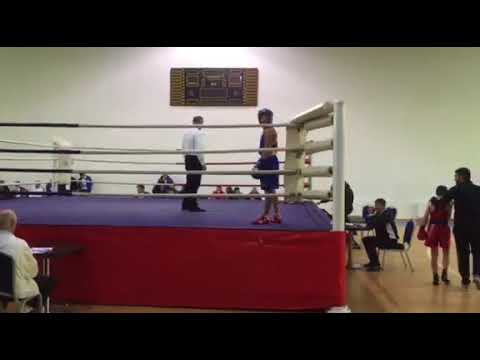The image depicts a vibrant scene inside a gymnasium, focused around a boxing ring set on a shiny hardwood floor. The foreground features a boxer clad in dark shorts, a helmet, and boxing gloves, standing in the right corner of the ring. To his right is a referee dressed in a white long-sleeved shirt and black pants. The boxing ring itself has a red exterior and a blue mat, enclosed by white posts and horizontal ropes alternating in black and white towards the middle. In the background, the gym is abuzz with activity: spectators are seated, possibly judges, and people are milling around, including a noticeable pair—a parent, with an arm around a child in a red uniform and matching boxing gloves, walking away from the ring. A white wall adorned with an unreadable sign and a scoreboard completes the backdrop of this evidently amateur boxing event.